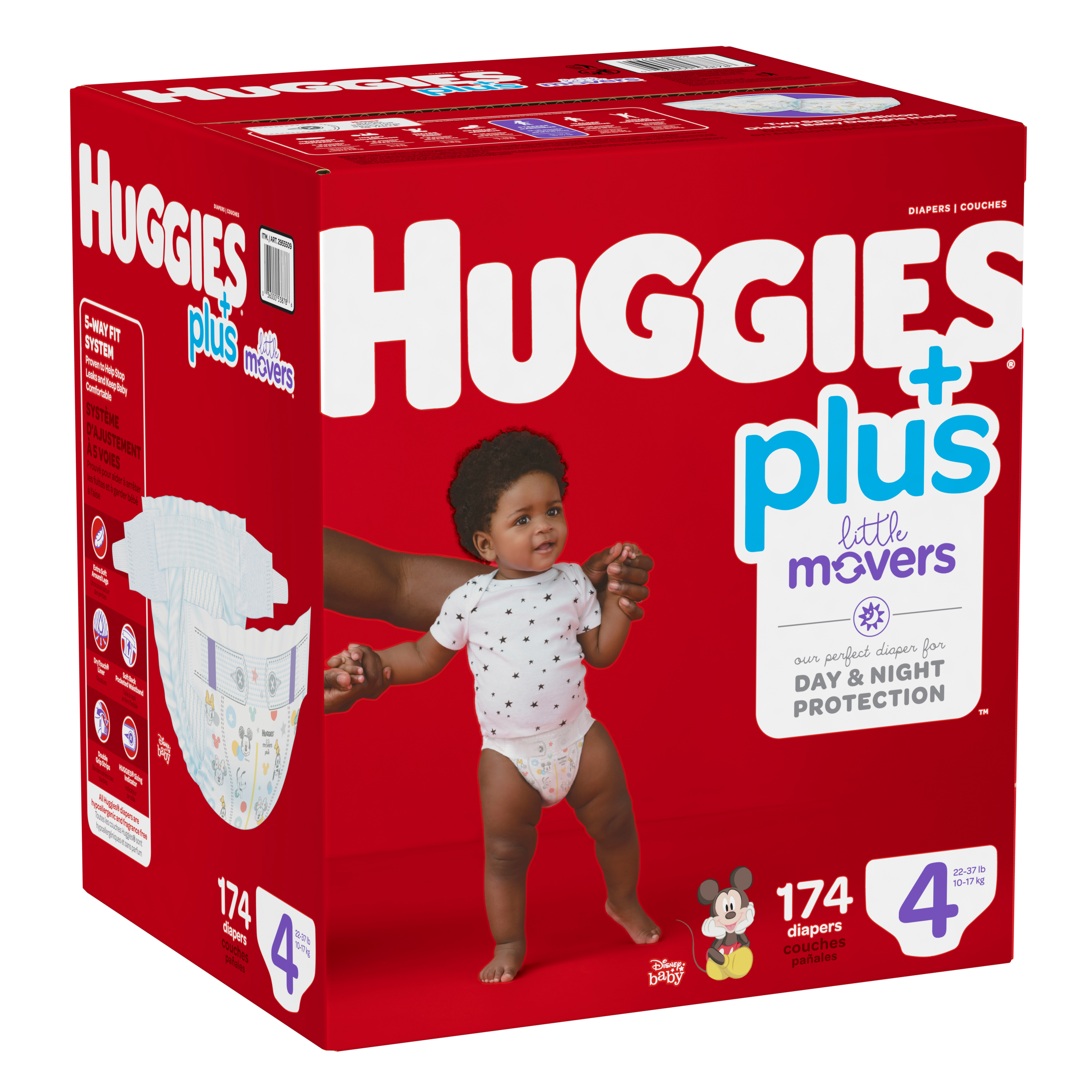This image captures an angled view of a red box of Huggies Plus Little Movers diapers set against a clean white background. Dominating the top portion of the box is the white Huggies logo, while the word "Plus" appears in light blue on the side. Centrally featured is an image of a young black baby with short curly black hair, dressed in a white onesie patterned with dark purple stars, and barefoot. The baby is standing up with the support of adult hands, likely depicting a parent. Additional text on the box reads "Little Movers: Day and Night Protection" in both purple and gray font beneath an icon of a sun and crescent moon. In the bottom right corner, an image of Mickey Mouse is accompanied by text stating "174 diapers, size 4". Near this, detailed product benefits such as "5-Way Fit Stretch" are depicted in diagrammatic circles. Further advertising details, including kilograms and pounds, and additional Spanish text frame other portions of the package. Light reflections and shadows give depth to the box's surfaces and details, offering a comprehensive view of the box's design and informational elements.